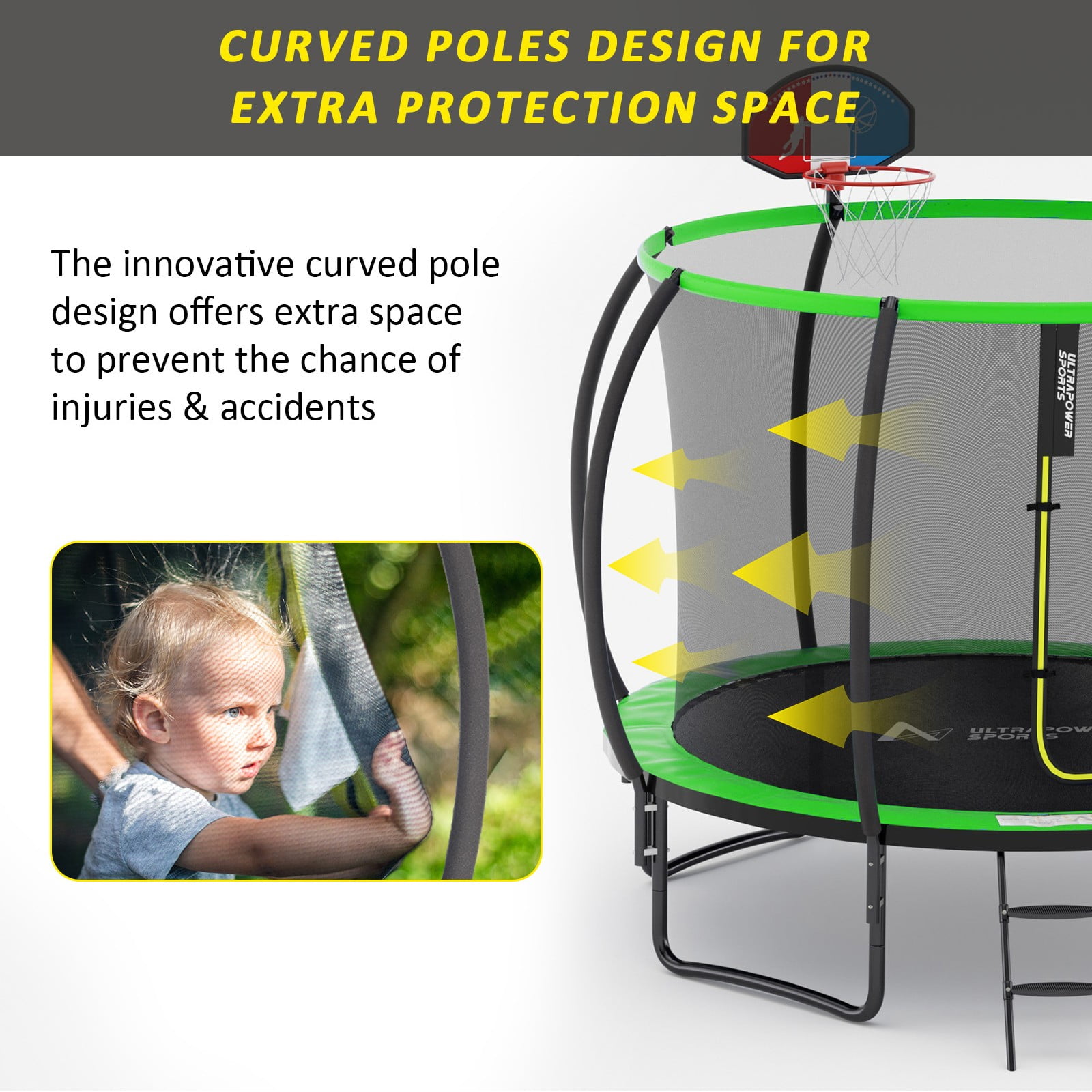The large square advertisement features a dark gray rectangular header at the top, with bold, all-caps yellow and white text stating "CURVED POLES DESIGN FOR EXTRA PROTECTION SPACE." Below this is a white and light gray background, against which a left-aligned paragraph elaborates on the benefits of the product: "The innovative curved pole design offers extra space to prevent the chance of injuries and accidents."

Central to the image is a rectangular photo depicting a young blonde-haired, blue-eyed boy touching a bar or object. Positioned on the right side of the image, there is a large trampoline with a surrounding net for safety. The trampoline, supported by metal bars and featuring a small metal ladder, is highlighted with neon green at both the top and bottom. A series of large yellow arrows point towards the left, emphasizing the protective netting that encloses the trampoline and prevents falls. The trampoline also includes a red, white, and blue basketball hoop at its center, adding an extra element of play.